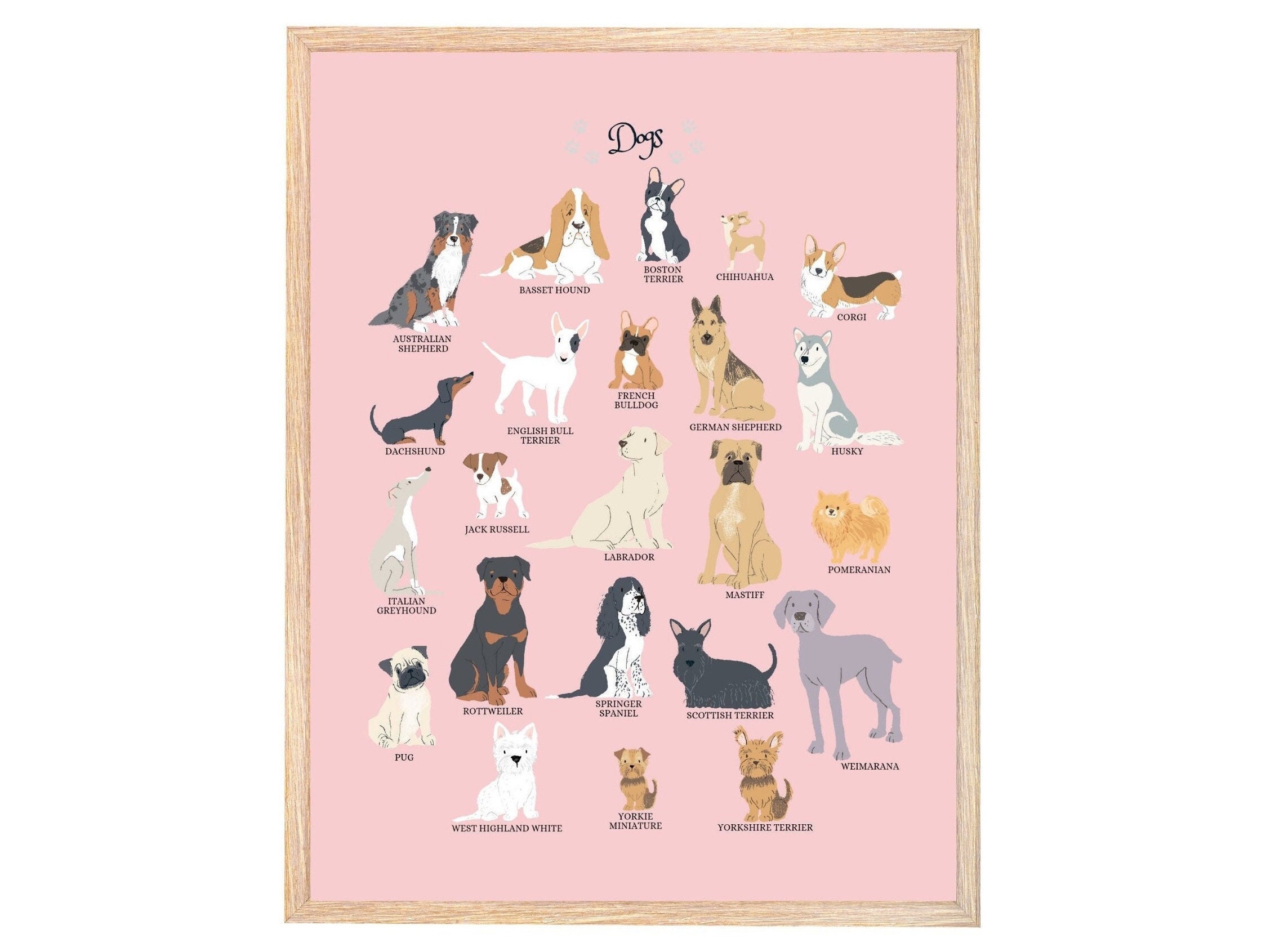This framed digital artwork features a vibrant, cartoon-style illustration titled "Dogs" in bold black text at the top. It showcases 23 dog breeds intricately drawn against a pink background, with each breed meticulously detailed to highlight their unique characteristics. The breeds include: Australian Shepherd, Basset Hound, Boston Terrier, Chihuahua, Corgi, Dachshund, English Bull Terrier, French Bulldog, German Shepherd, Husky, Italian Greyhound, Jack Russell, Labrador, Mastiff, Pomeranian, Pug, Rottweiler, Springer Spaniel, Scottish Terrier, Weimaraner, West Highland White Terrier, Yorkshire Terrier, and a Yorkie Miniature. The dogs are evenly distributed in rows of five, except the bottom-most row, which has three. The illustration captures a variety of colors and features such as long and short ears, diverse nose shapes, different leg lengths, and various tail types, ranging from long to short to none. Completing the composition is a wooden frame that encloses the artwork, providing a finished, polished look.